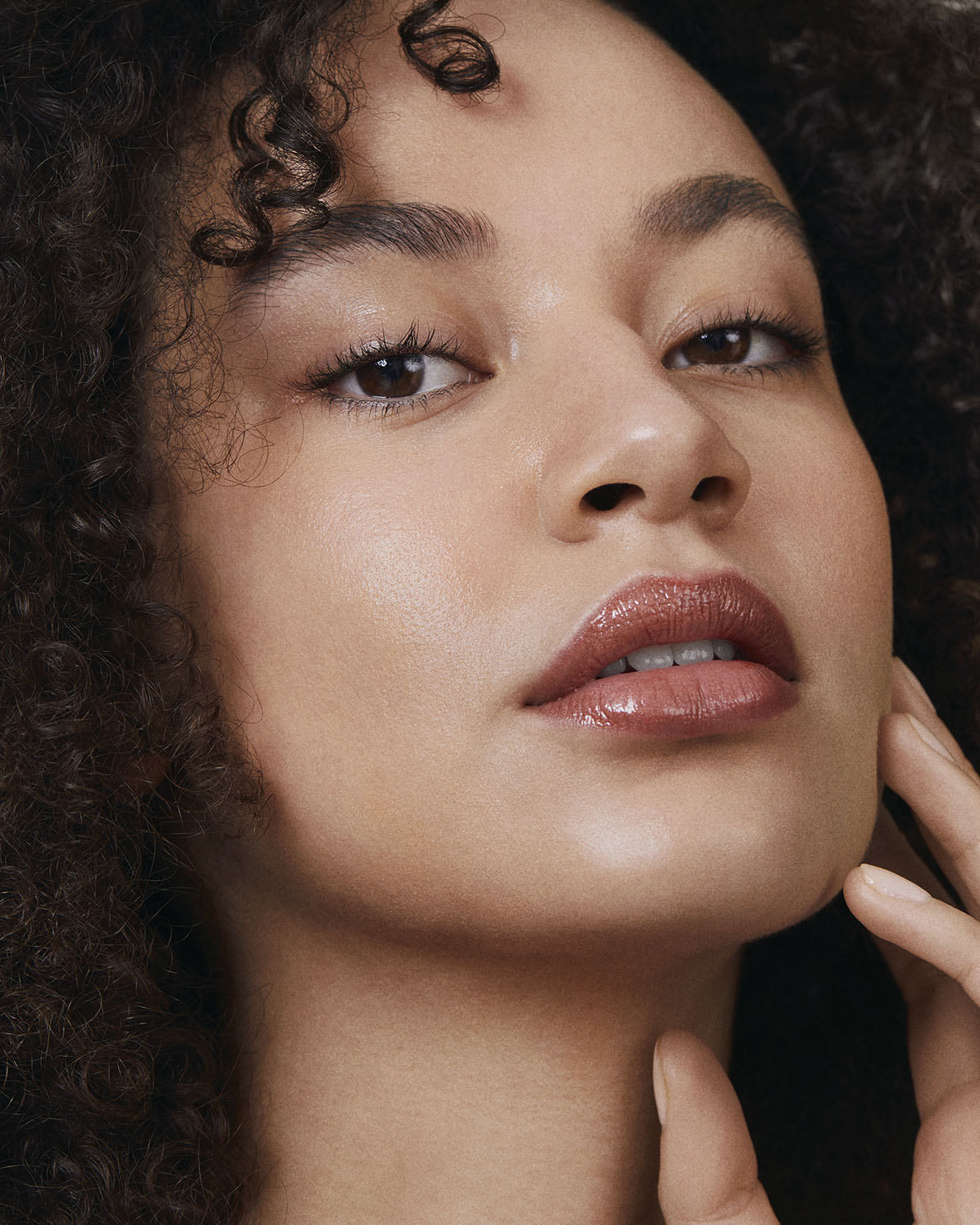The photograph is a close-up glamour shot of an attractive young woman, intended for use in TV, film, or modeling. The image captures her head and neck, with her face slightly tilted upwards and turned towards the right. She has striking black curly hair that falls around her face, some curls even touching her forehead. Her well-defined, dark eyebrows and dark brown eyes are accentuated by makeup, including notable mascara. She has a soft shine on her smooth, medium-brown skin, particularly on her cheeks, eyelids, lips, and chin, giving her complexion a flawless look. Her lipstick is a muted red, and her mouth is slightly open, revealing the top row of her teeth. She holds her right hand up to her face, with her fingers gently touching her chin and her thumb resting in front of her throat, adding an element of allure to the pose. Her fingernails appear to have a very light pink polish. The lighting, coming from the upper right, highlights her features perfectly, enhancing the overall dramatic and captivating effect of the photograph.